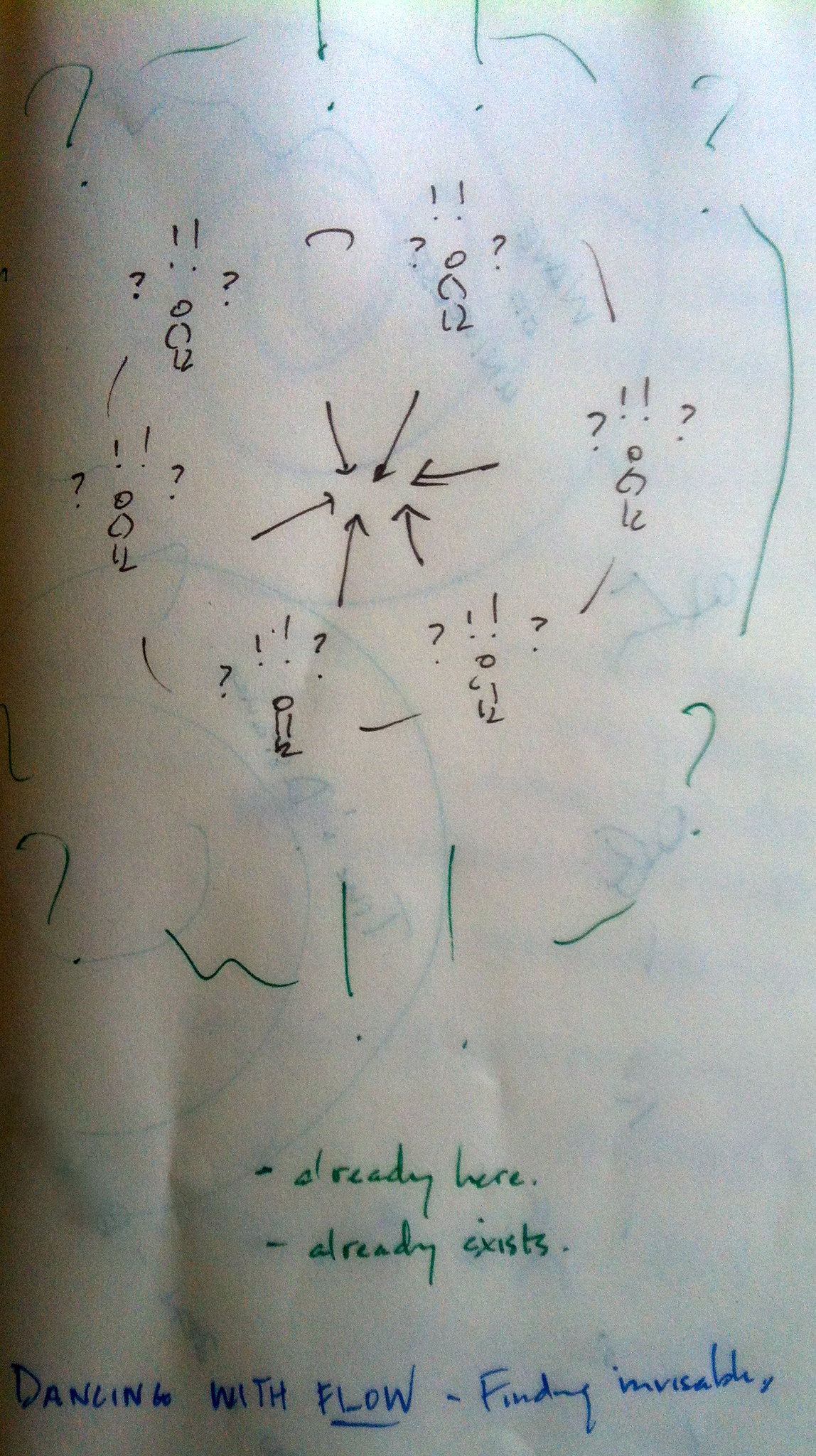The image depicts a large, white, glossy sheet of paper prominently displayed. The paper is covered with an array of intricate markings and numbers. At the bottom, there are two small dashes in green ink; one is labeled "already here," and the other is labeled "already exists." Additionally, the phrase "dancing with flow" is written in bold blue letters, with the word "flow" underlined.

Further details include a series of two lines descending from the top, leading into an area resembling a cloud-like formation at the center. Surrounding the central formation, typical clock positions—such as where 2, 4, 7, and 9 would be—are marked with question marks instead of numbers. Within this perimeter, smaller marks include a combination of "0 0 4," question marks, and exclamation points spread throughout, resembling tiny footprints.

Concentrically within these markings, there is an intricate pattern, and at the very core of the arrangement, six black arrows converge, all pointing towards the center of the circle, drawing the viewer's focus to this focal point.